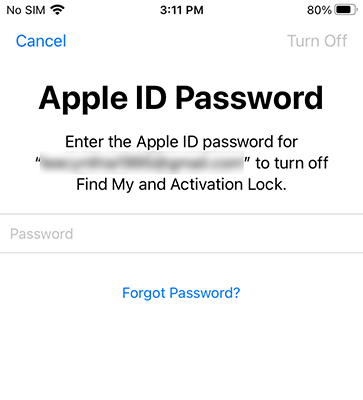Screenshot Description: 

This screenshot, taken from an Apple iPhone, captures a notification screen regarding the Apple ID password. 

At the top left corner, the status bar displays "No SIM" along with the wireless signal indicator. Centered at the top is the current time, "3:11 PM." The top right corner shows the battery level at "80%" with an accompanying battery icon partially filled to indicate the charge status.

The main title, prominently displayed in bold black letters, reads "Apple ID Password." Below this title, the text instructs the user to "Enter the Apple ID password for," followed by a space where the user's personal information, now blurred for privacy, would appear. 

The text continues, stating, "To turn off Find My iPhone and Activation Lock," with each initial letter capitalized for emphasis. Two grayscale lines are present at the bottom section, adding to the overall style and layout.

On the bottom left, grayed-out placeholder text reads "Password," indicating where the password should be entered. Amidst the grayscale elements, a blue hyperlink stating "Forgot password?" is positioned at the bottom center of the screen, offering a way for users to retrieve their password if necessary.